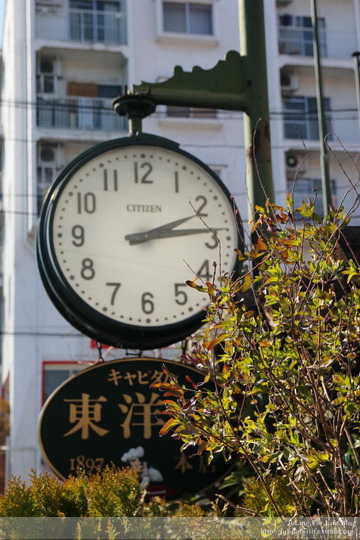A classic clock with Arabic numerals, displaying the time as approximately 2:14, hangs from an ornate metal frame outside an apartment building. Below the clock, there's a sign adorned with Asian characters and partially obscured by greenery, with the number "1897" visible. The scene is brightly lit by the sun, although the building's facade is in shadow, indicating the sun is on the opposite side. A barely legible credit mark is positioned in the bottom right corner of the image.